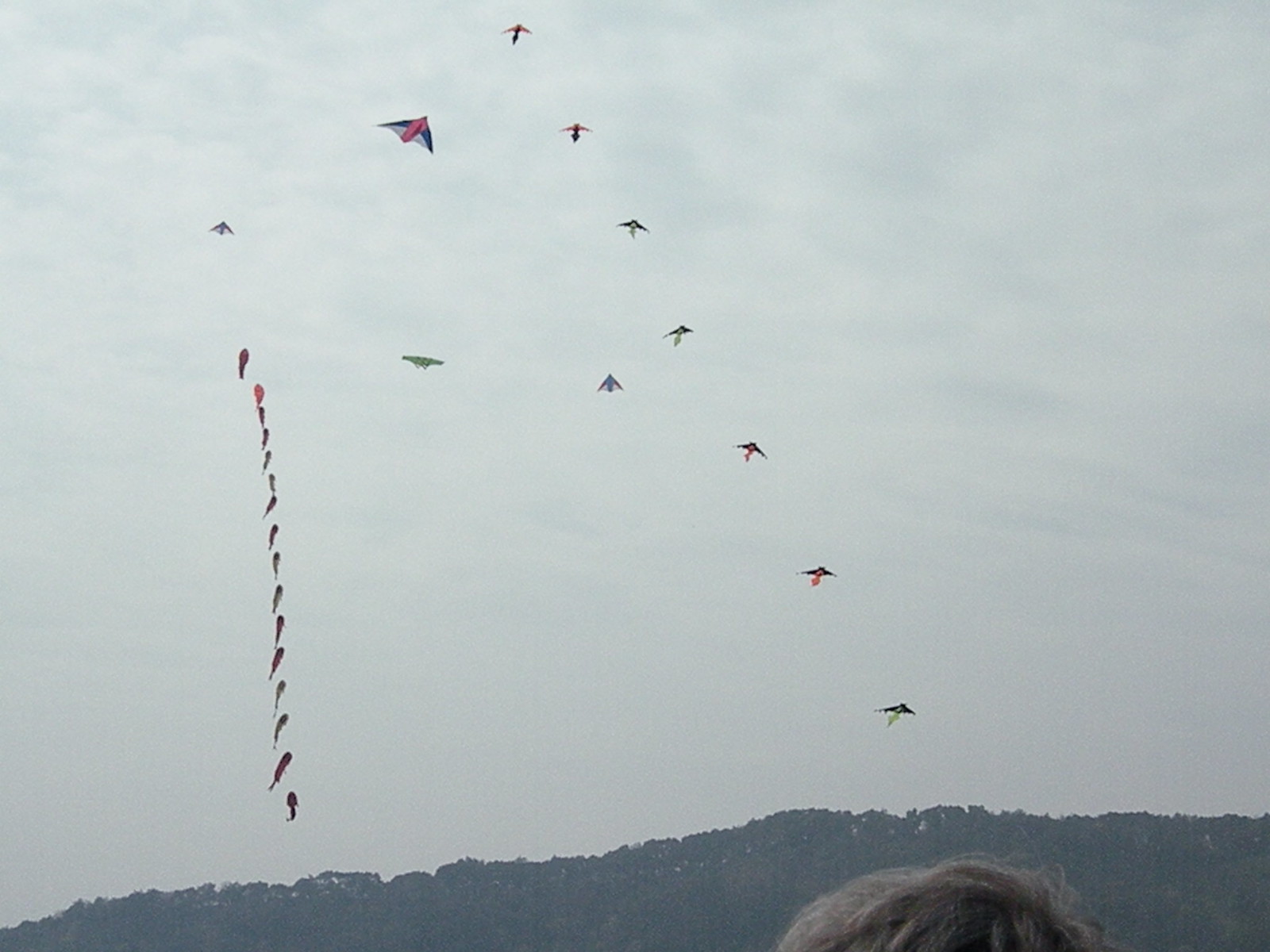On a very cloudy and muted grey day that looks like it's about to rain, an array of vibrant kites are flying in the sky outdoors. The far background is filled with grey-tone trees and faint mountains at the bottom edge of the image. The kites form two distinct lines: one vertical row on the left-hand side ascending upward, and another diagonal line. These kites include a variety of colors: blue, red, blue and white, green, pink, red and black, green and black, and orange. Among them, a green kite stands out in the middle. In the bottom right-hand corner of the image, the top of someone's brown hair is visible, adding a human element to this dynamic and colorful kite-flying scene.